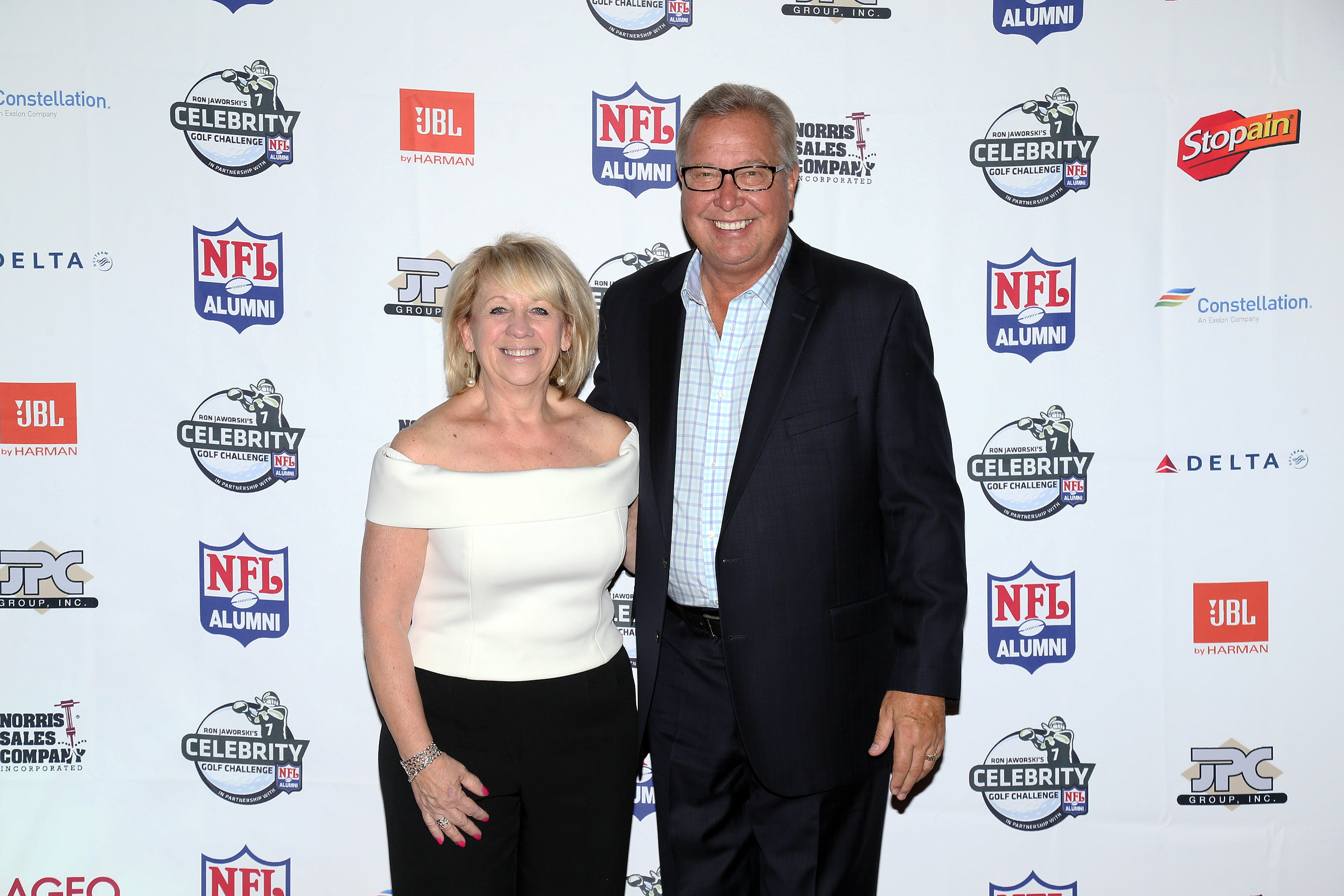In this photograph, an older couple, likely in their 60s, stands in front of a backdrop featuring various company logos and event inscriptions, prominently including the NFL Alumni Association and references to a Celebrity Golf Challenge, hinting at a golf tournament for retired NFL players and celebrities. 

The man, positioned on the right, is notably taller than the woman. He is wearing a dark blue suit with an open jacket and a light blue shirt adorned with a dark blue square pattern. His broad smile, black plastic-rimmed glasses, and short gray hair complement his Caucasian appearance. The woman, standing to his left, gives a classic, stylish appearance in a manila off-the-shoulder top and black pants. She accessorizes with a silver bracelet and simple earrings, and her shoulder-length blonde hair frames her broad smile. Both individuals appear delighted to be photographed at this event, exuding happiness and warmth.